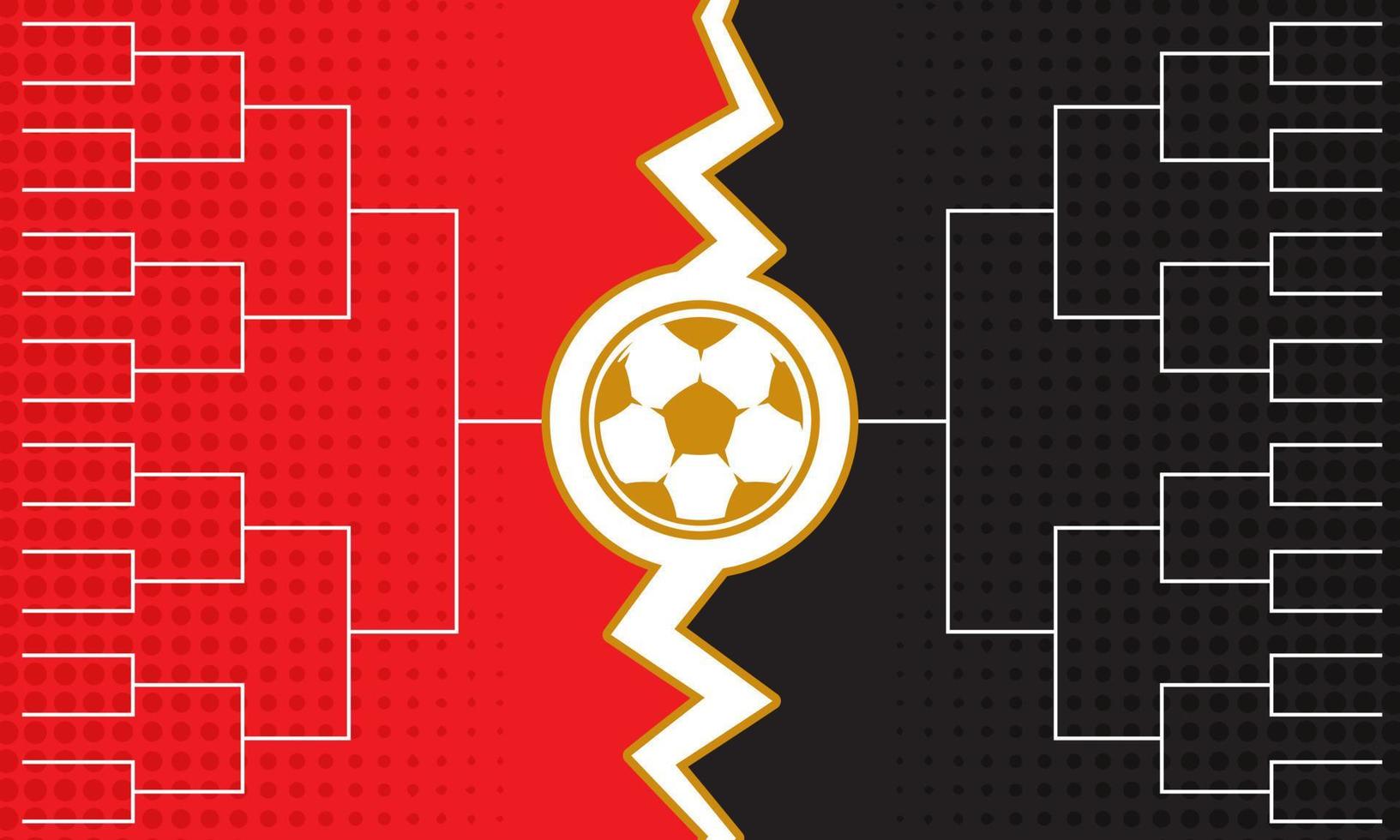This minimalist illustration represents a soccer tournament bracket template. The design features a gold and white soccer ball at the center, with a dynamic white and gold lightning bolt stretching vertically through the ball, symbolically dividing the two sides. The left half of the image is marked with a red background adorned with darker red polka dots, while the right half mirrors this with a black background and even darker black dots. Both sides of the bracket are designed to host 16 teams each, leading to the final matchup at the center. The colors utilized are strictly red, black, white, and a light brown-gold color, creating a bold yet simple visual. The overall design is clean and empty, ready for team names to be added as the tournament progresses.